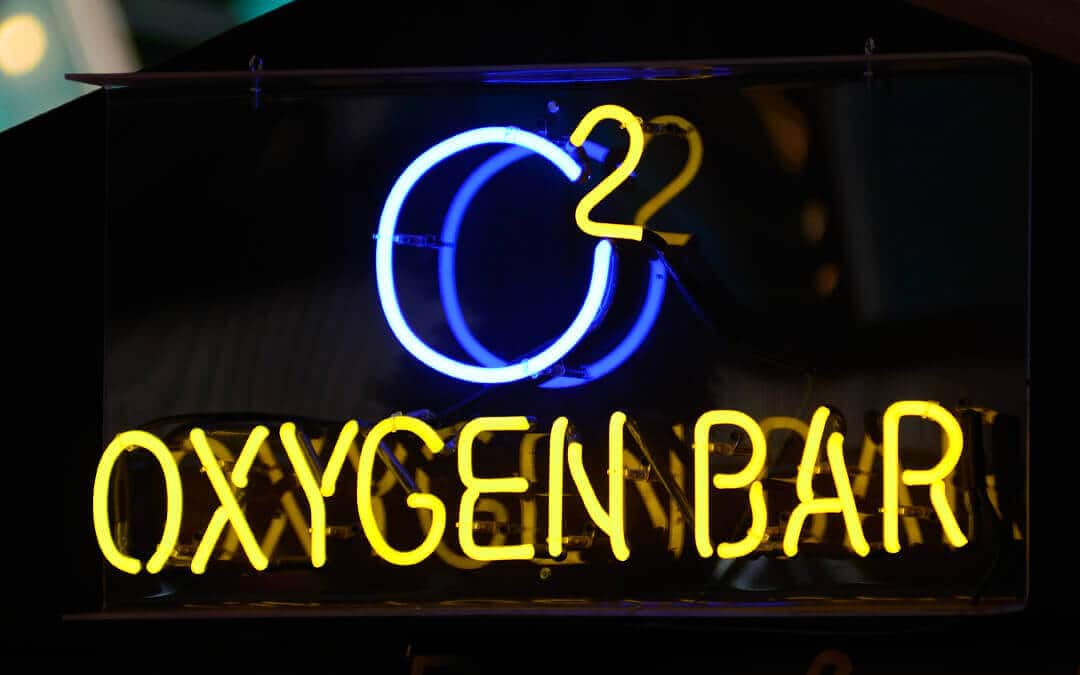This image features a neon sign for an oxygen bar. At the top, the sign displays "O2" where the 'O' is in a white or bluish light blue neon, accompanied by a dark blue reflection behind it. The '2' is in a bright yellow neon. Beneath the "O2" lies the text "oxygen bar," also in yellow neon, with a yellow reflection behind it. The entire sign appears to be encased in glass, with a small black line and two hooks on each side at the top. It's set against a black background, giving it a striking contrast and making the neon colors pop. In the top left corner, there is a blurry trace of a white or yellow circle and line, possibly suggesting a moon or another light source in the distance. The setting appears to be outdoors at night, enhancing the vividness of the neon lights. This oxygen bar sign beckons from the darkness, inviting visitors to step inside for an O2 experience.